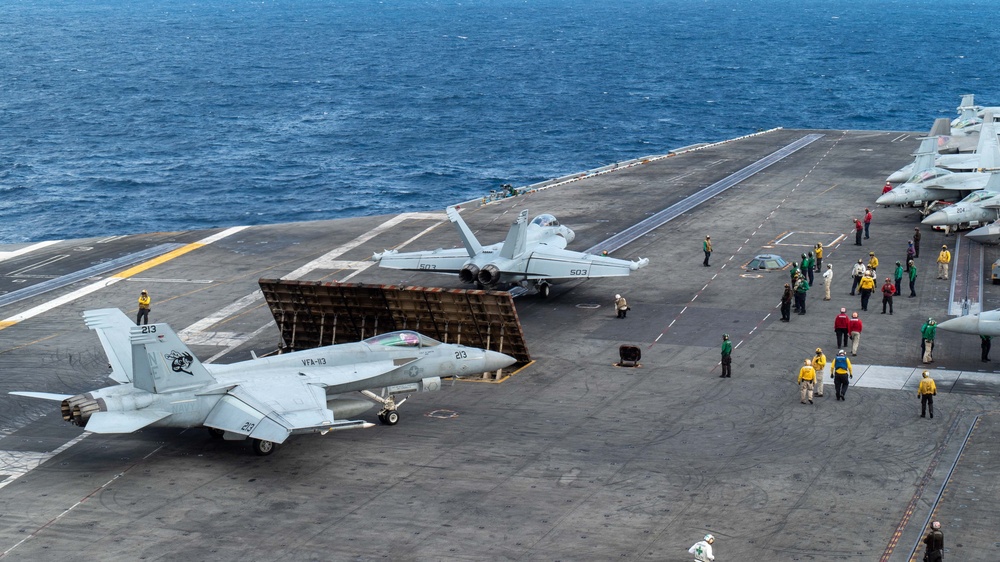A vibrant photograph captures an aircraft carrier at sea, against the backdrop of a blue ocean. The focus is on the bustling flight deck, where an intense launch operation is underway. Dominating the left side of the image, two fighter jets are poised for action; one is on the runway, ready to take off, while another waits just behind it, bearing the number "213" and featuring distinctive markings including "VFA-R3" on the upper fin. A man stands on the tail fin of this waiting jet, contributing to the dynamic scene.

The deck brims with activity: approximately 20 people are visible, each clad in colorful attire signifying their roles—yellow, green, red, white, and black tops reflect a spectrum of ranks and duties. Some personnel are actively preparing the jets for launch, while others observe the proceedings or move about the deck. The man in the center of the picture, donned in an orange shirt and black pants, adds to the colorful mosaic.

The right side of the image is lined with additional fighter jets, about half a dozen to eight, neatly arranged in a queue, their noses pointing westward. These jets, similar in style and uniformly white, are stationed on a concrete surface marked with white and yellow lines, delineating the bustling, organized chaos of a naval flight deck.